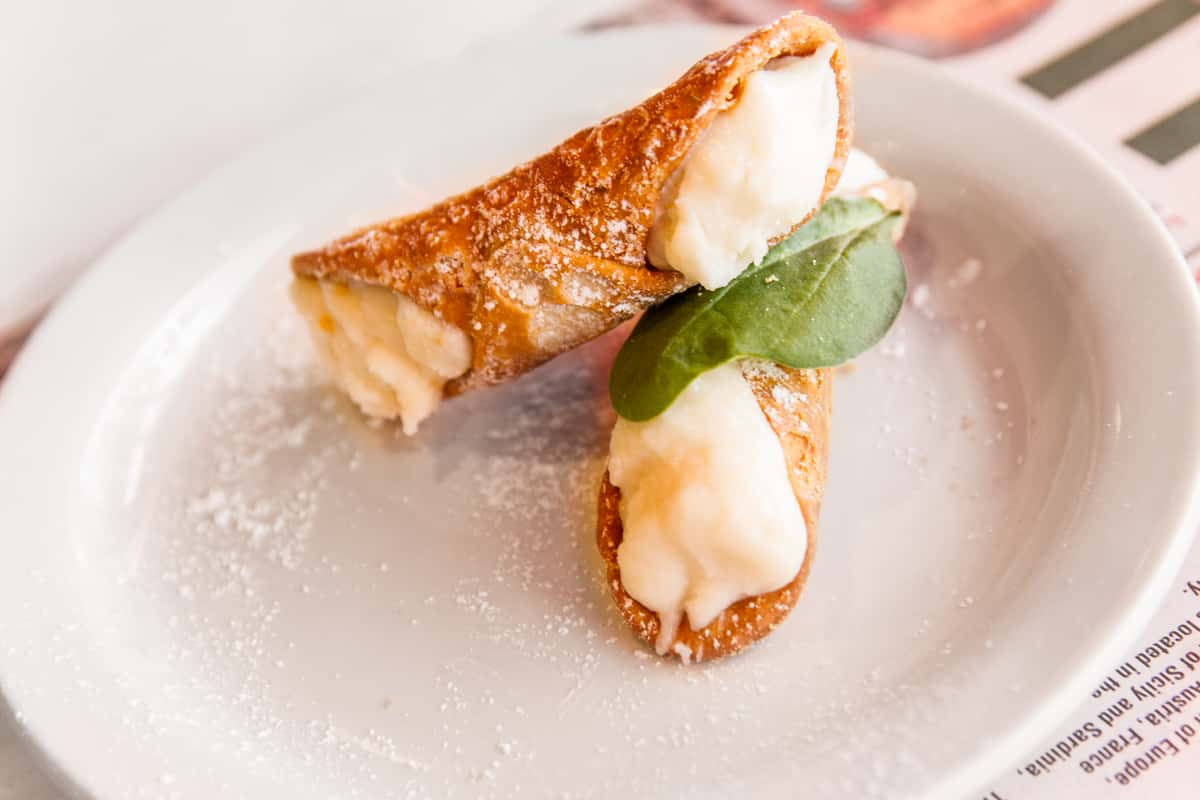The photograph features two Italian cannoli desserts placed on a white, round plate, which rests on a table covered with a white tablecloth adorned with green stripes. The crispy, brown shells of the cannolis encase a creamy, yellow filling. One cannoli leans on top of the other, and a green leaf serves as a garnish, positioned between the two pastries. The plate is lightly dusted with powdered sugar. Additionally, a piece of white paper with English text can be seen in the bottom right corner of the image, adding a subtle contextual detail.